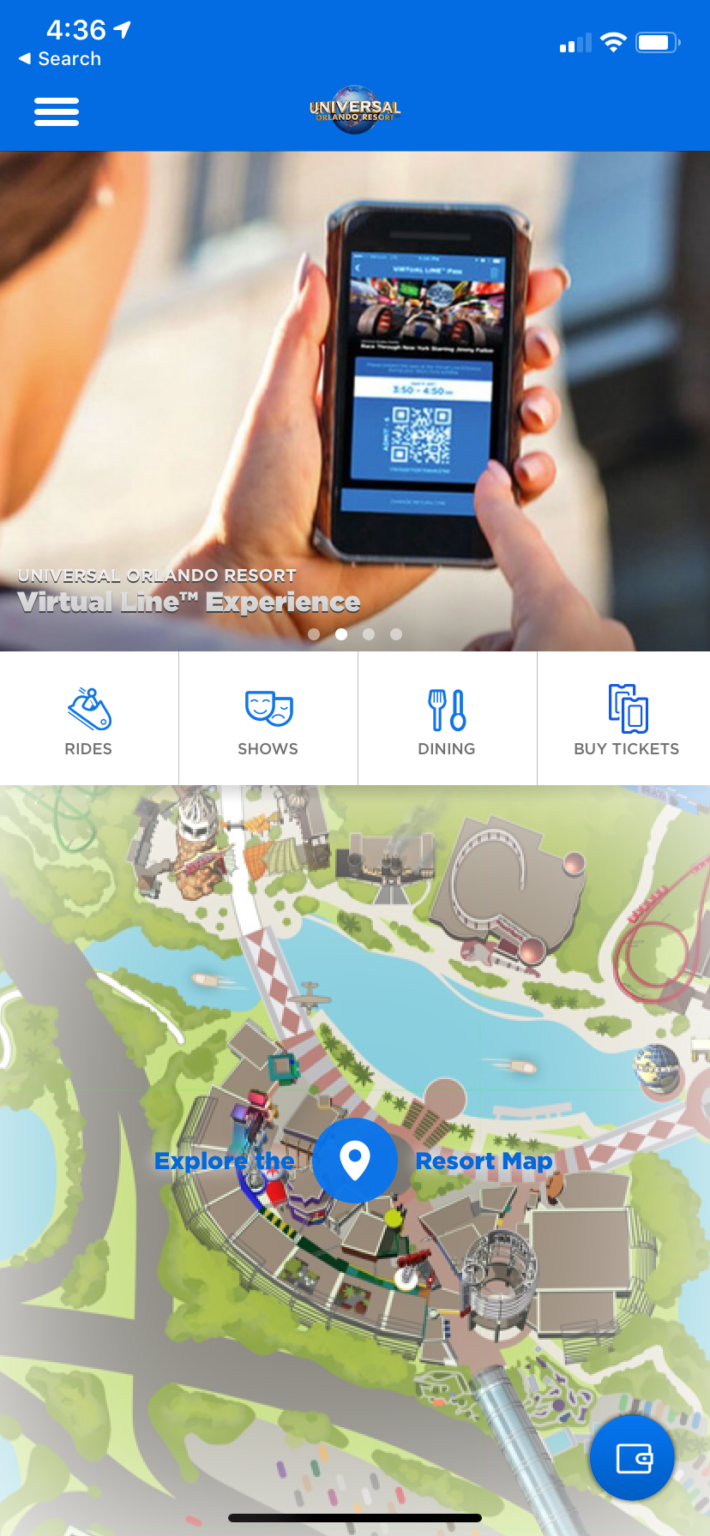This image showcases a screenshot of a mobile application with a blue horizontal rectangle spanning the top part of the screen. In the upper left-hand corner, the white text displays the time along with a send arrow icon. On the upper right-hand side, reception, Wi-Fi, and battery indicators are clearly visible. 

Beneath the time on the left, there's a left-pointing arrow resembling a sideways triangle, accompanied by a small "Search" label. About two lines down, a white hamburger menu icon appears, centrally flanked by the Universal logo.

The prominently featured photograph centers on the back of a woman's head as she holds a cellphone in her hand. Superimposed on the photo is text promoting the "Orlando Resort Virtual Experience."

Below the photograph, there are three interactive buttons with blue icons and gray text, separated by thin vertical gray lines. These buttons are labeled sequentially as: "Rides," "Shows," "Dining," and "Buy Tickets."

Further down, a detailed map of the resort is displayed. On the right side, it says "Resort Map," while the left side features an "Explore" option. A blue location icon marks the center of the map, which illustrates various buildings, water features, and green grassy areas.